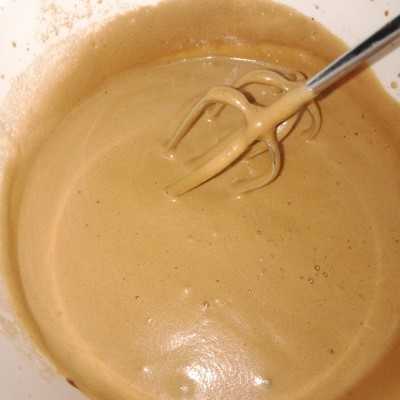The image depicts a close-up view of a mixing bowl filled with a creamy, caramel-colored batter or potentially a brownish sauce. Inside the bowl, two silver, shiny chrome hand mixer attachments with four-pronged blades each are immersed in the thick liquid, actively stirring it. The pronged mixer blades are designed with two blades coming from the front and two from the side, ensuring thorough mixing. The edges of the bowl show residue from the batter, indicating it has been well-mixed. The bowl and its contents occupy most of the image, suggesting the setting is likely a kitchen, although no additional kitchen elements are visible. The creamy substance against the white border of the bowl contrasts with light to moderate tan shades, highlighting the mixing process.